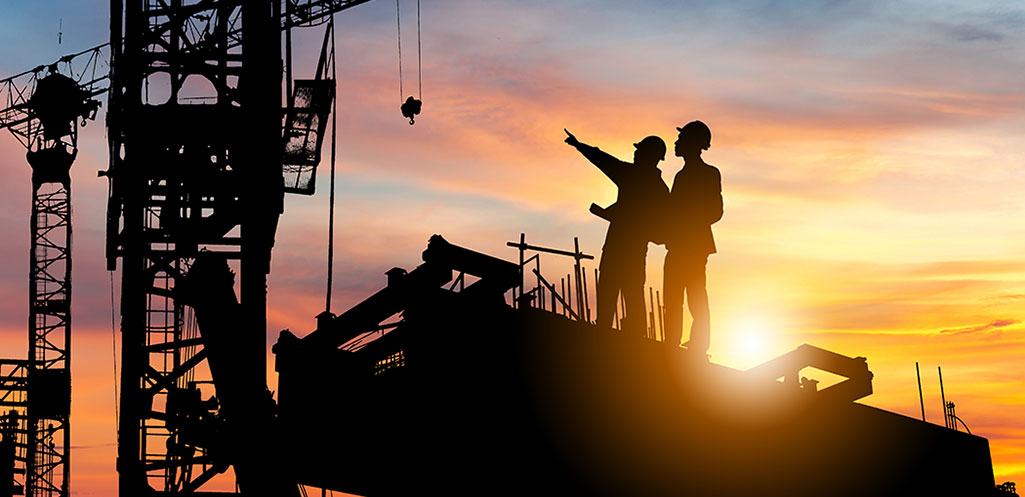In this detailed image taken at sunset, the sky is painted in warm hues of orange and pink, with the sun setting low on the horizon and clouds adding a vivid touch to the scenery. The main focus is on two men standing on a black metal scaffolding at a construction site, both wearing protective helmets. Positioned prominently on the left side is a tall crane, extending from the bottom left to the top left of the frame. The men, only visible as silhouettes, are side by side in the middle of the shot, engaged in conversation. One man stands slightly ahead of the other, his left arm extended and pointing towards the crane. They are surrounded by upward-arching rebars and other construction equipment, adding to the industrial setting of the photograph.